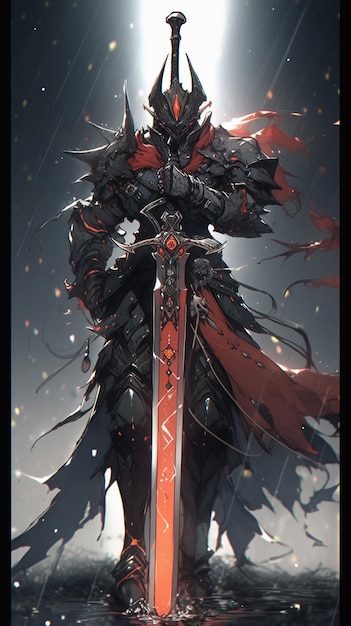This digital illustration portrays an imposing knight-like figure, reminiscent of a character from a video game such as Skyrim, captured in a dramatic and compelling pose. The figure stands in the foreground, clad in intricate black armor accented with dark brownish-red hues and red details. The knight is adorned with a dark cape and bears prominent horn-like structures atop its helmet, which features an orange, diamond-shaped marking on the forehead. Positioned facing directly towards the viewer, the knight holds a large, elaborately designed sword, thrust firmly into the ground. An aura of intensity is evident with the glowing red sword that appears almost molten in the middle.

Surrounding the figure, the environment is shrouded in darkness, pierced by a striking white light that backlights the knight, casting dramatic shadows and creating a sense of mystique. This luminous backdrop could be interpreted as a stormy sky or a stark light from an opening, adding to the enigmatic atmosphere. Additional subtle details include possible skull motifs on the knight's waistband and intricate designs on the sword and red accents on the clothing. With the knight possibly setting foot in water amid a rainy scene, the image masterfully combines sharp, edgy artistry with a rich color scheme dominated by black, red, and interspersed with yellow highlights. The overall effect is a compelling, sharply rendered portrait of a formidable, almost mythical warrior.